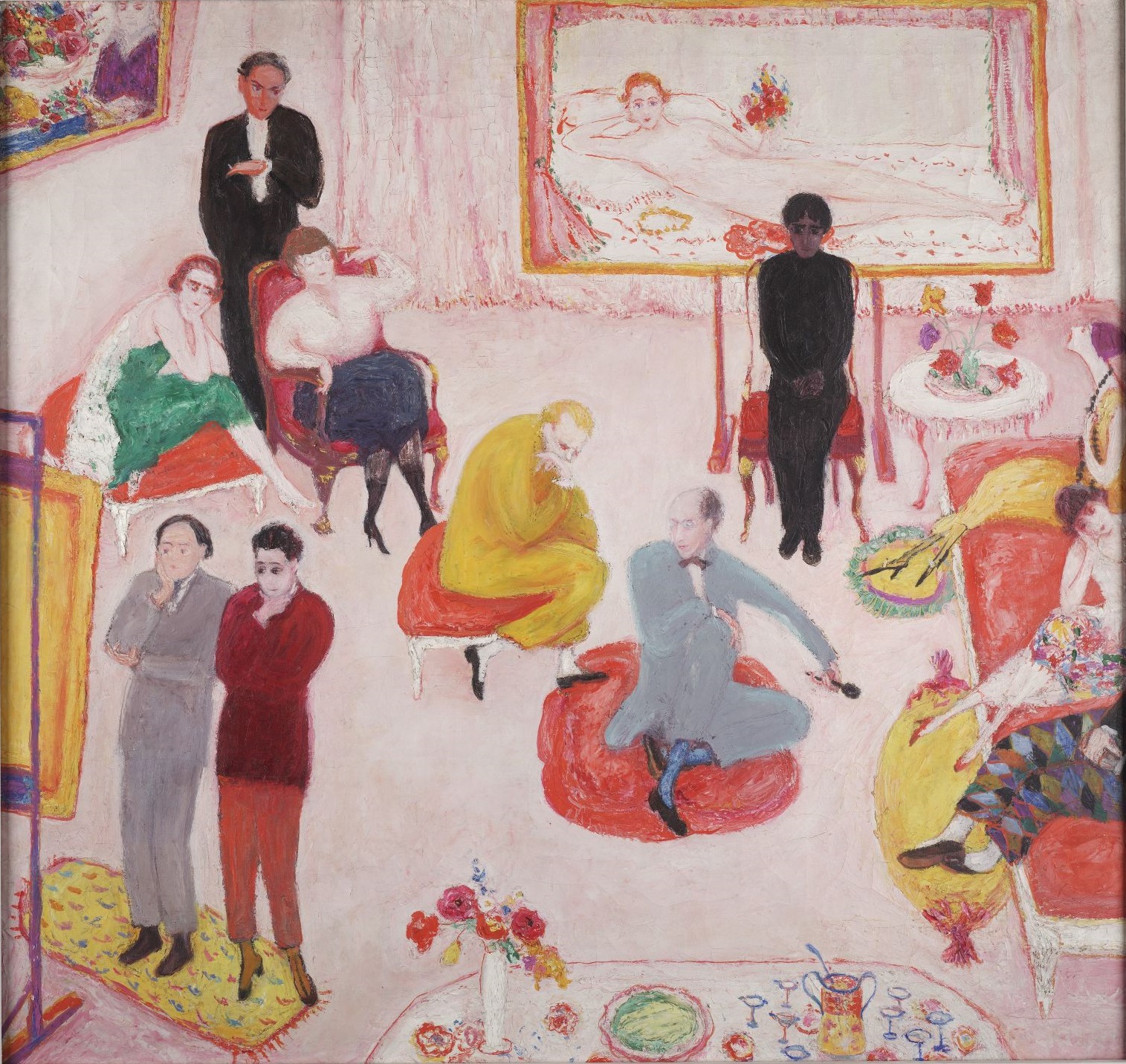The painting depicts a scene in a room, possibly a parlor or an art gallery, characterized by an early 20th-century style reminiscent of Chagall. The composition is two-dimensional with a unique perspective, showcasing a predominantly pink backdrop with red and pink furniture. Among this setting are around ten people, engaging in quiet conversation or contemplation, many appearing rather bored.

On the left, two men stand with their hands on their faces—one in a gray suit and the other in a red top. Nearby, a table adorned with flowers contributes to the room's vibrant ambiance. The center features men in yellow and gray suits, engaged in conversation, against a backdrop of vividly colored paintings. One prominent painting along the left wall displays purple, pink, blue, and yellow hues, while a stark, softly colored painting of a nude woman reclining on a chaise lounge dominates the back wall.

In various spots in the room, people are seated on red chairs, cushions, couches, or stools. To the left, a woman in a green dress converses with another in a blue skirt and white blouse. On the long red couch to the right, three ornately dressed women are seated. Interspersed among these individuals are others, some standing and some sitting, all adorned in brightly colored attire including red, gray, and black suits, contributing to the rich, vivid palette of the painting. The entire scene is enveloped in hues of red, pink, black, yellow, green, and blue, inviting viewers into its somewhat surreal, whimsical atmosphere.